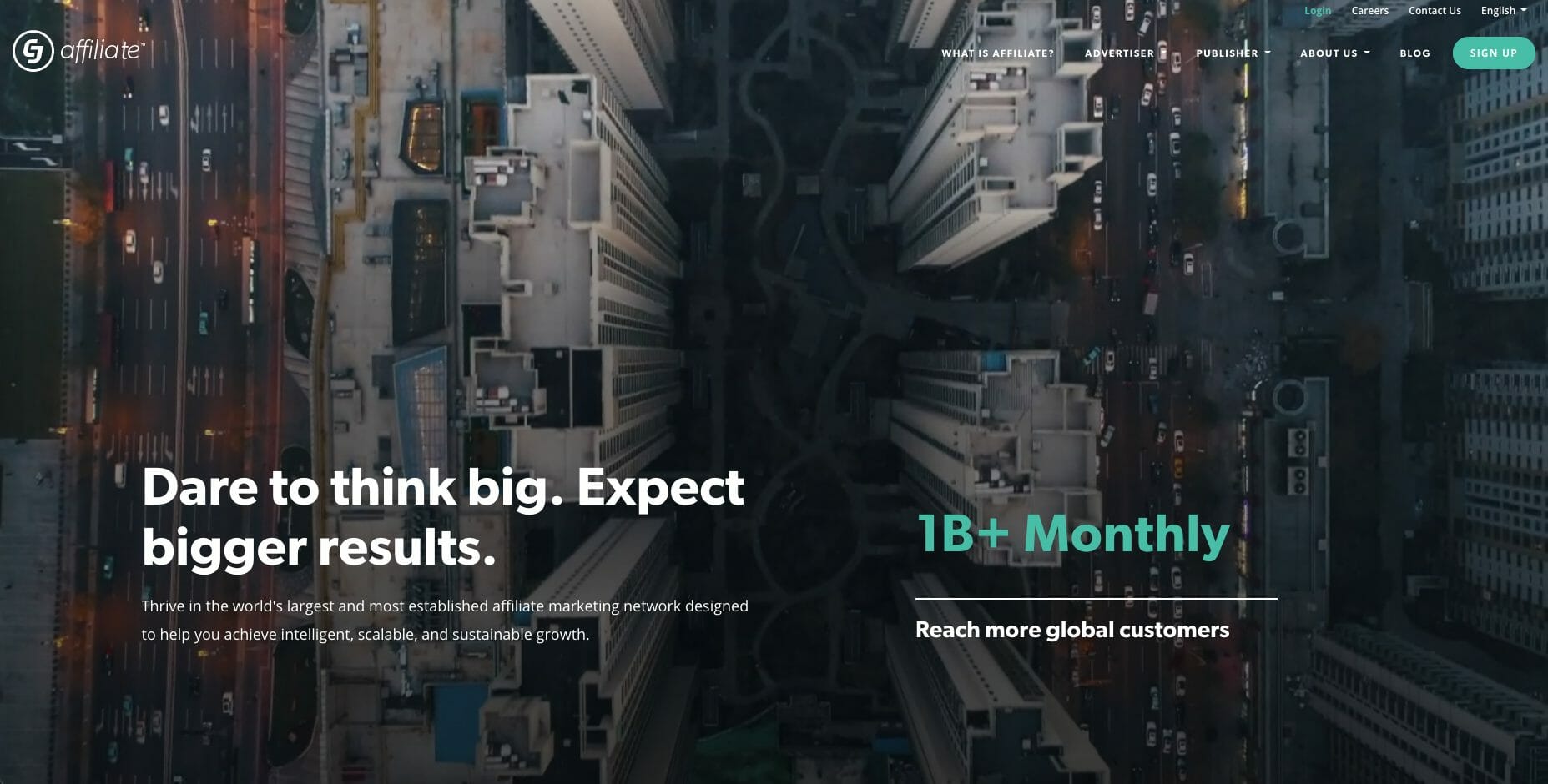The web page showcases an intricate design with a professional feel, starting at the top left corner with a distinctive icon resembling interconnected letters 'C' and 'J' wrapped in a circle. Adjacent to this icon, the word "affiliate" is displayed in a sleek, white lowercase font. To the right of this branding, a small navigation menu appears, consisting of options such as "Login," "Careers," "Contact Us," and "English," all in diminutive font size.

Beneath this navigation are additional links arranged horizontally: "What is Affiliate," "Advertiser," "Publisher," "About Us," and "Blog." Also included is a prominent green button emblazoned with the call-to-action "Sign Up" in white text.

A central section of the page features bold, eye-catching text in white that reads, "Dare to think big. Expect bigger results." Below this motivational headline is a descriptive subtext: "Thrive in the world's largest and most established affiliate marketing network, designed to help you achieve intelligent, scalable, and substantial growth." Complementing this message, the right side of this section highlights statistics in green font, notably "1B+ monthly," with an encouraging statement underneath in white font: "Reach more global customers."

The entire textual content overlays an expansive cityscape image, depicting towering skyscrapers and various tall buildings. To the left side of the image, a bustling street with cars driving up and down adds dynamism to the urban backdrop.